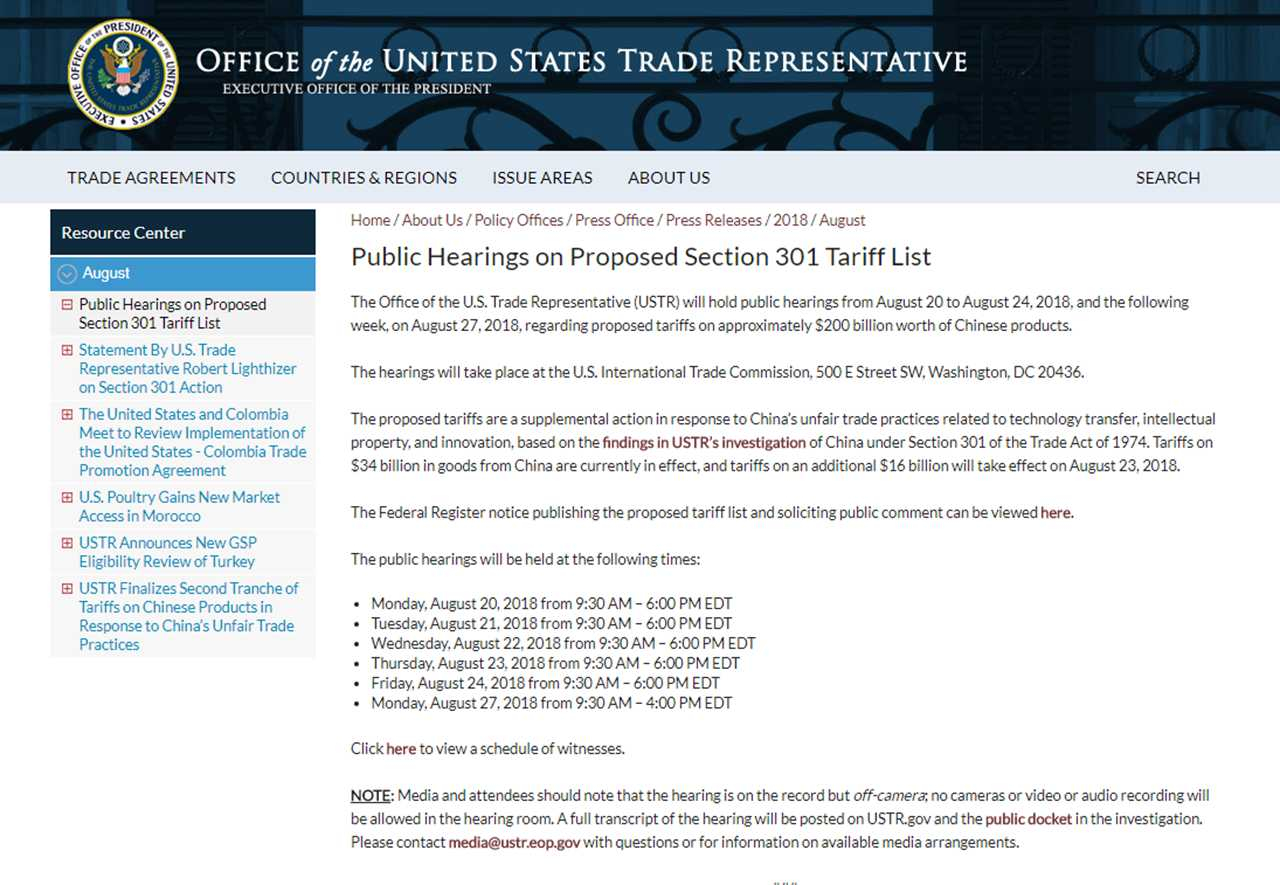The screen capture showcases the official website of the Office of the United States Trade Representative, part of the executive office of the President. Dominating the top section is a dark blue banner, adorned with an intricate image of wrought iron work. Centered on this banner, and rendered in crisp white text, is the office's title. Adjacent to the text, on the left, proudly sits the Presidential Seal: a blue circle outlined in white, featuring a bald eagle gripping a cluster of arrows in one talon and an olive branch in the other, with the iconic American flag crest centered on the eagle’s chest.

Beneath this prominent banner, a gray navigation bar offers seamless access to various sections of the website, labeled as "Trade Agreements," "Countries & Regions," "Issue Areas," "About Us," and "Search." The left side of the page features a vertical navigation menu, utilizing shades of gray, blue, and black, with text mainly consisting of blue, clickable links.

The main content area of the page combines a white background with black text. The current page focuses on "Public Hearings on Proposed Section 301 Tariff List," a header that stands out in bold black font. Below this header, several paragraphs detail the specifics, followed by a bulleted list outlining six scheduled dates and times for the public hearings. Additional information for the media and attendees is noted at the bottom, ensuring comprehensive coverage of this section.